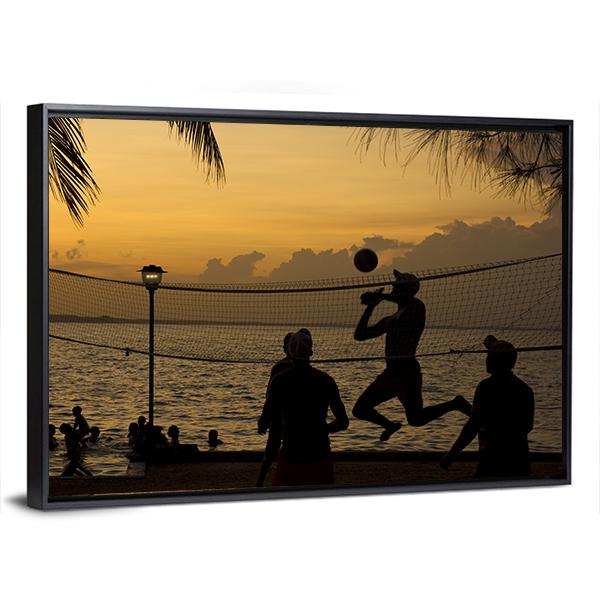This image features a computer-generated, framed artwork with a sleek, three-dimensional black rectangle frame. Inside the frame, it captures the dynamic silhouettes of four people engaged in an exhilarating game of beach volleyball. One player is prominently seen leaping into the air, poised with the volleyball near his face, ready for a powerful strike. The other three players, also silhouetted, gaze intently upwards, tracking the ball's trajectory. The backdrop showcases an idyllic beach setting with gentle waves extending out into the horizon where a group of silhouetted people enjoy the water in the bottom left corner. A black light pole stands prominent near this group. This spirited scene unfolds against a stunning sunset sky, painted with rich hues of orange and interspersed with wisps of clouds. The upper portion of the image is adorned with silhouettes of tree leaves, adding a touch of nature to this animated tableau.